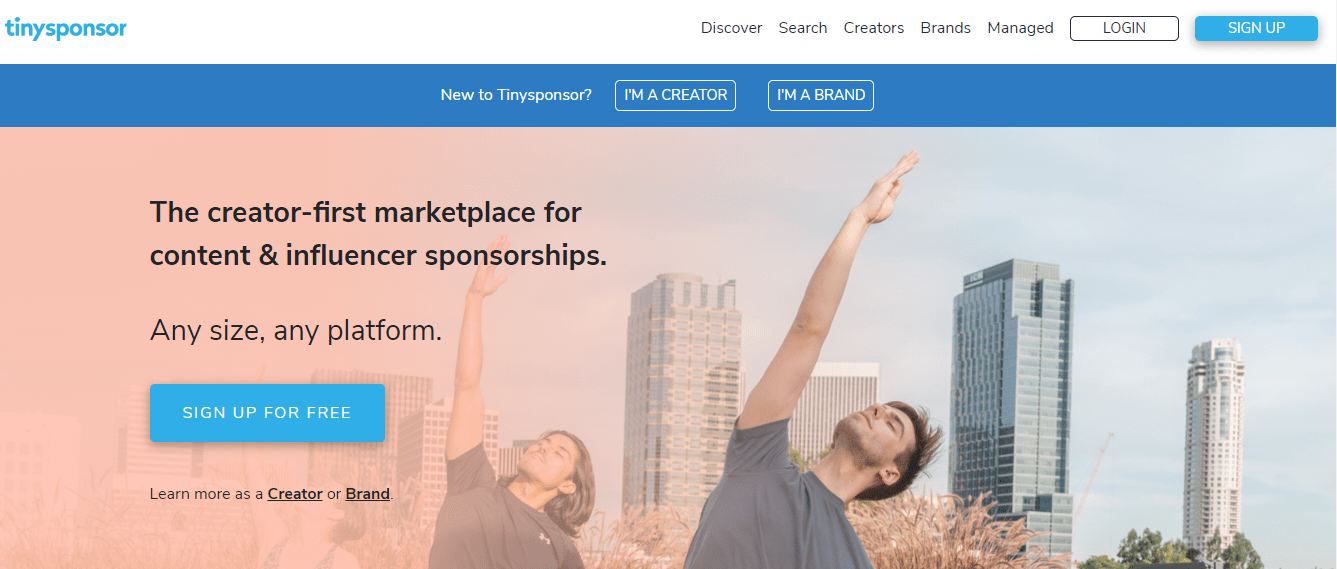Screenshot of the Tiny Sponsor Homepage:

At the top left corner of the image, "Tiny Sponsor" is prominently displayed in blue text against a clean white background. The navigation links are neatly aligned on the right-hand side, from right to left: Sign Up, Log In, Managed, Brands, Creators, Search, and Discover.

Directly below the navigation bar, a striking blue banner with white text asks, "New to Tiny Sponsor?" and features two interactive buttons: "I'm a creator" and "I'm a brand."

The main section of the screenshot is dominated by a wide, engaging graphic depicting two people engaged in exercise with a dramatic skyscraper backdrop. Both individuals are captured mid-movement, their arms lifted skyward and bent at an angle, adding a dynamic feel to the visual.

To the left of this graphic, a bold message is printed in black ink on a beige background: "The Creator First Marketplace for Content and Influencer Sponsorships. Any size, any platform." Below this impactful statement, a prominent blue button encourages action with the text "Sign Up for Free."

Finally, at the bottom of the section, small black text invites further exploration with underlined phrases: "Learn more as a creator" or "brand."